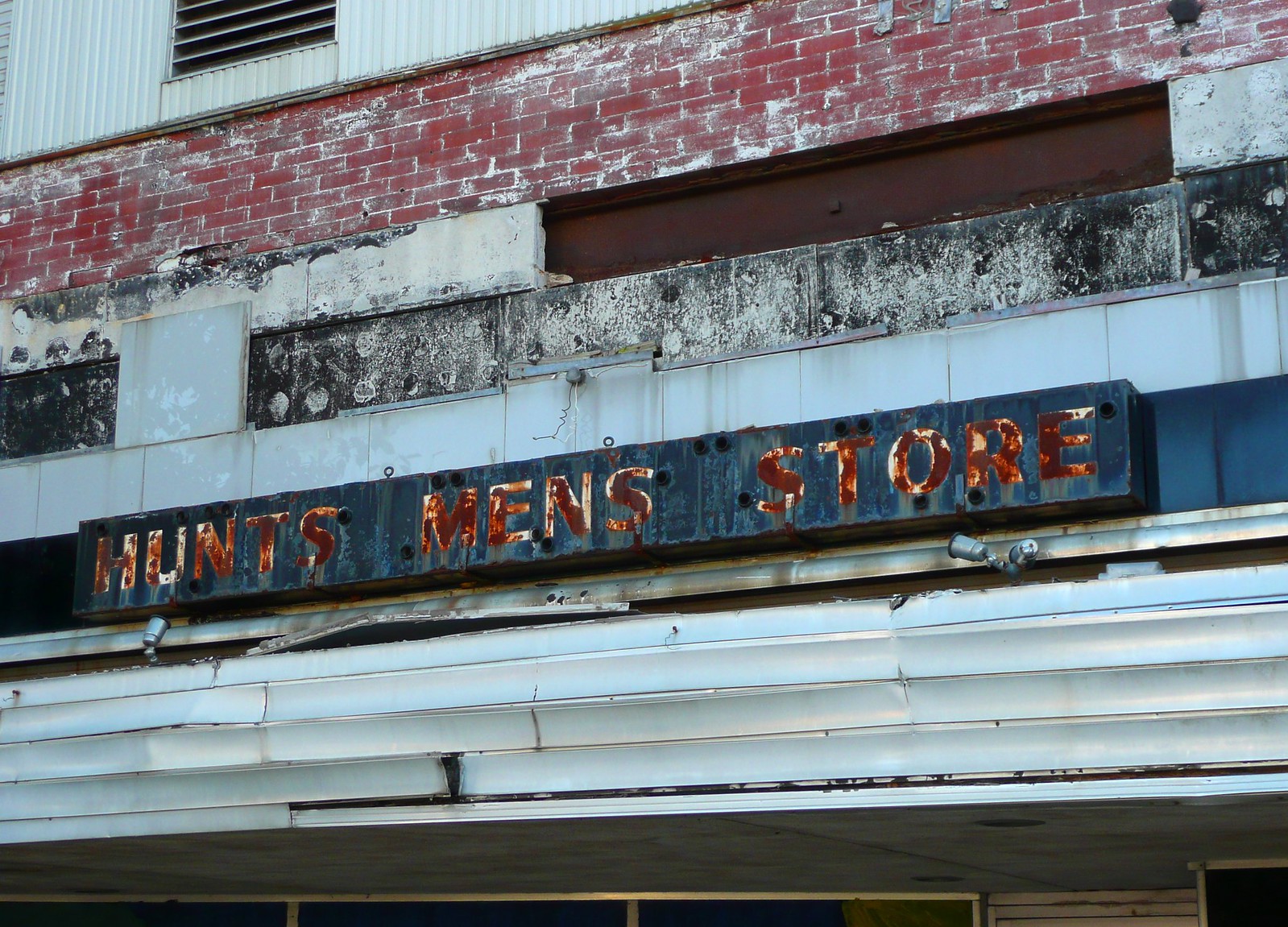This image captures a highly distressed store sign for "Huntsman's Store," prominently featured in faded blue with nearly illegible white letters now dominated by rust. The sign, which once proudly marked the establishment, is severely weathered, revealing rusty brownish and reddish hues that mar its surface. Positioned beneath the sign is a series of white poles, increasingly deteriorated and dented, transitioning from brownish-grayish to spots of white. Above the sign, a section of dilapidated black tiles, some missing, is visible, further highlighting the worn state of the structure. Additionally, there's an indication of red brickwork marred with white blotches, denoting significant aging and exposure to the elements. Corrugated plastic sheets line the upper part of the wall, providing stark contrast to the otherwise vintage and rustic appearance. At the base of the image, a glimpse of shutters or gutters in white is seen, alongside a doorway, suggesting the entrance to the store.